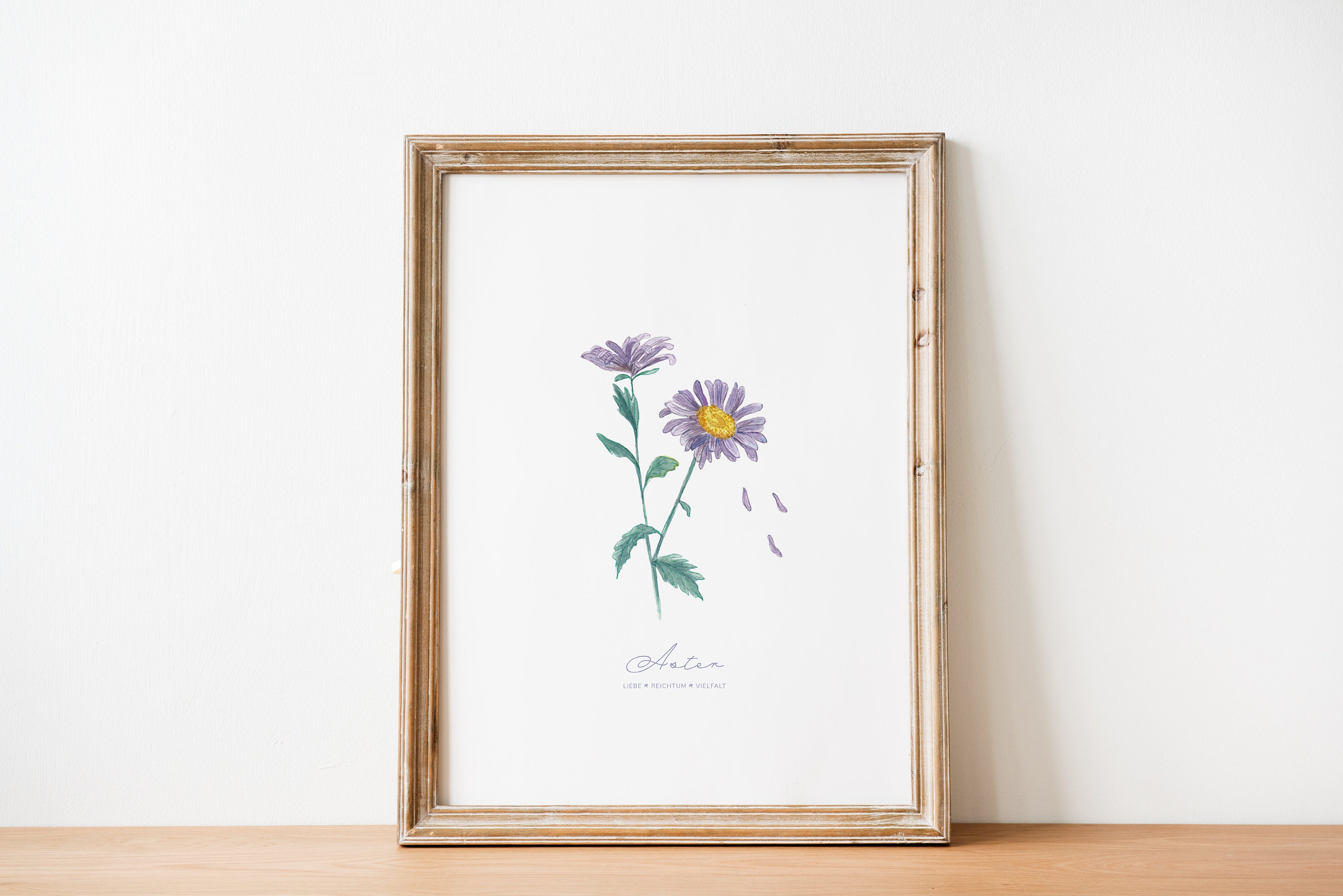The photograph captures a picture in a frame, leaning against a pristine white wall. The frame is made of very light wood with subtle white streaks, exuding a muted golden hue. The framed picture rests on a surface that appears to be either a very light wood table or floor. Central to the artwork within the frame are two purple daisies on a white background. The daisies are connected by a green stem, eventually merging into a single stem. The left daisy features three leaves, while the right one has two large leaves and one very small leaf. Notably, three petals from the left daisy appear to be gently falling off towards the ground. Below the flowers, there's cursive and printed text, likely a signature and additional wording, which remains too small to decipher. The overall composition is clean and elegantly simple, highlighting the soft beauty of the flowers and the delicate artistry involved.